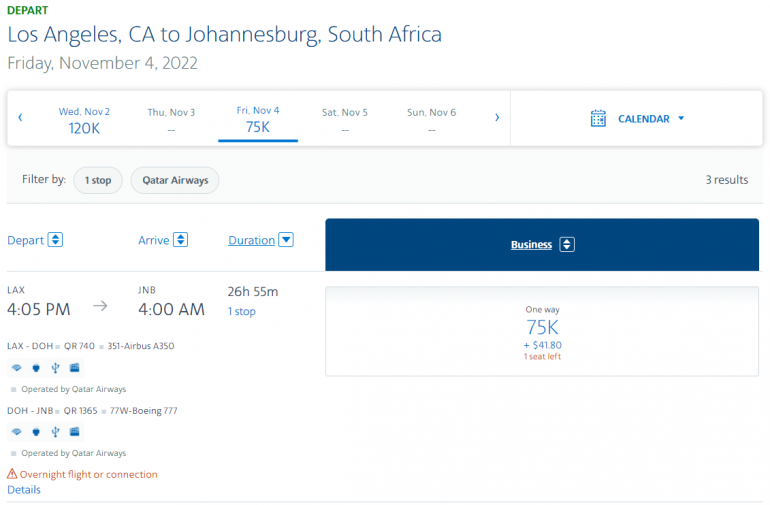The image displays detailed flight information on a white background. In the upper left corner, the word "Depart" is prominently highlighted in green. Below this, it indicates the flight route: "Los Angeles, California to Johannesburg, South Africa," with the departure date listed as "Friday, November 4, 2022." 

A blue-highlighted bar underneath features "Wednesday, November 2, 120K" and "Friday, November 4, 75K," with the latter highlighted in blue as well. To the right, there is a blue calendar dropdown for date selection.

Scrolling down, users can filter flights by criteria such as "one stop" or "Qatar Airways." The interface also includes dropdowns for "Depart," "Arrive," and "Duration." On the right is a "Business" button, indicating the class of travel.

The specific flight details show a departure from LAX at 4:05 PM, arriving at JNB Airport at 4:00 AM, with a total flight duration of 26 hours and 55 minutes and one stop. The one-way fare is 75K miles plus $4,180. There's only one seat remaining.

Additional information confirms that the aircraft is a Boeing 777 ("77W"). A red notice indicates an "Overnight flight or connection." Users are prompted to click on "Details" for more information.